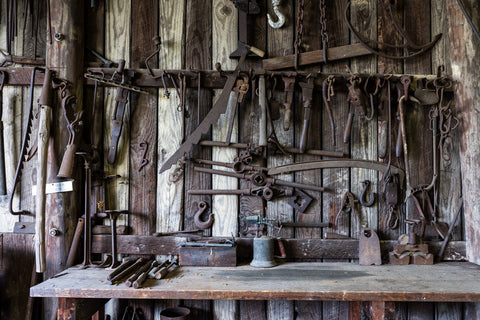This image depicts the interior of an old barn or shed, with walls crafted from alternating dark and light wooden planks. Dominating the left side is a sturdy vertical beam, attached to which is a crossbar supporting several hooks that hold a wide array of rusted, old-fashioned cast iron tools. The tools, which include saw blades, pliers, shears, shackles, clamps, and chains, evoke a historical atmosphere reminiscent of an 1800s workshop.

Below this rack of tools is a weathered wooden workbench. The bench stands on legs that are partially cut off at the bottom of the photo, with its surface cluttered with various items. Visible on the bench are a couple of hammers and canisters, along with pieces of metal and other objects being worked on. The bench appears dirty, with a noticeable wet spot in its center, further emphasizing the long-neglected state of this aged workspace.